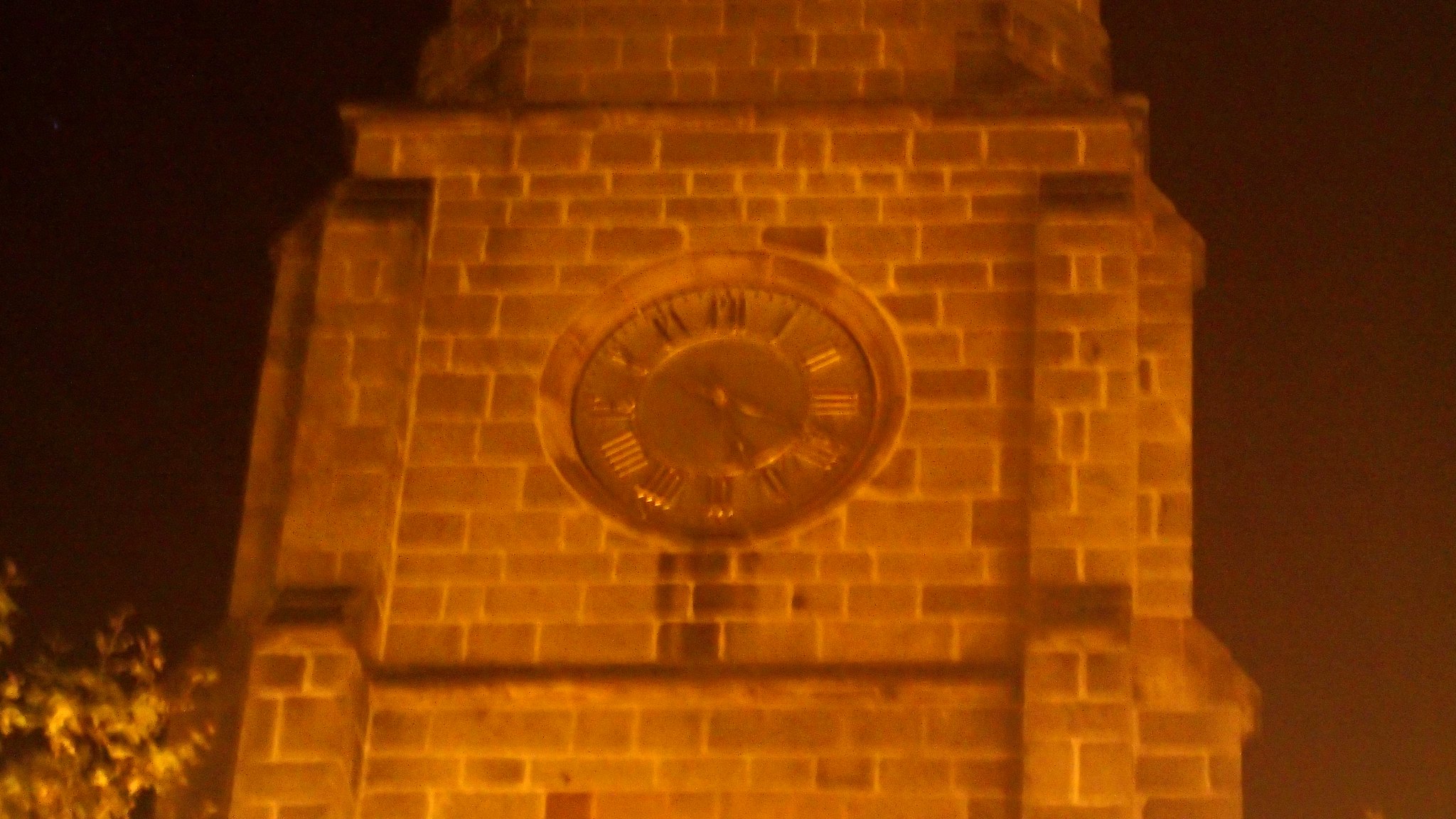A close-up nighttime image of a clock tower dominated by a monochromatic orange and rusty brown hue. The tower, built from either stone or dark-colored brick with white mortar, stands isolated in a pitch-black sky lightly tinged with red. The clock face, recessed into the middle of the tower, exhibits a metallic, bronze or brass appearance with clearly defined Roman numerals and hands, indicating 5:20 despite the darkness. The tower is illuminated from below, casting a dramatic light that skews the overall color palette and emphasizes the worn texture of the bricks. Additionally, the lower left corner of the image subtly reveals the tip of a bush or tree, adding a touch of nature to the stark architectural scene.